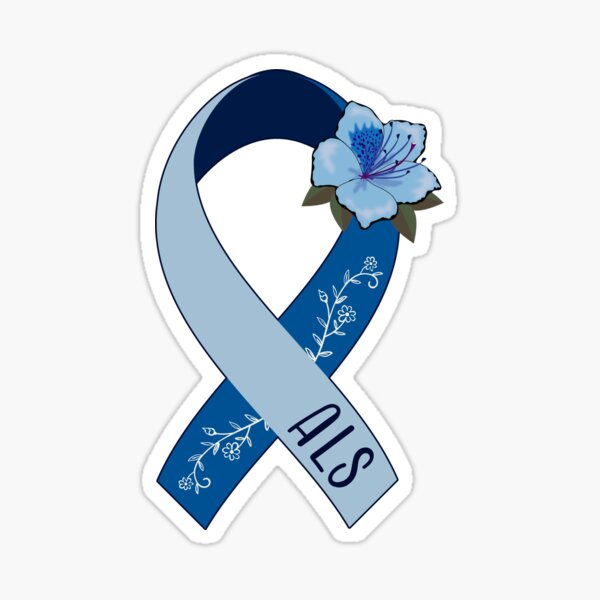The image is a hand-drawn illustration of a ribbon folded into the traditional awareness loop, with a design reminiscent of support ribbons commonly seen for various causes. This particular ribbon features a light blue and dark blue color scheme, with the text "ALS" prominently displayed on the light blue portion, signifying its association with ALS (Amyotrophic Lateral Sclerosis) awareness, also known as Lou Gehrig's disease. The ribbon is adorned with a delicate hibiscus flower near the center, colored in shades of blue with detailed purple stamens and green leaves, and an elegant vine or leaf motif running down its length. The illustration is set against a white background, emphasizing its suitability for printing on various mediums such as clothing, stickers, or magnets, potentially for fundraising or awareness events related to ALS research.